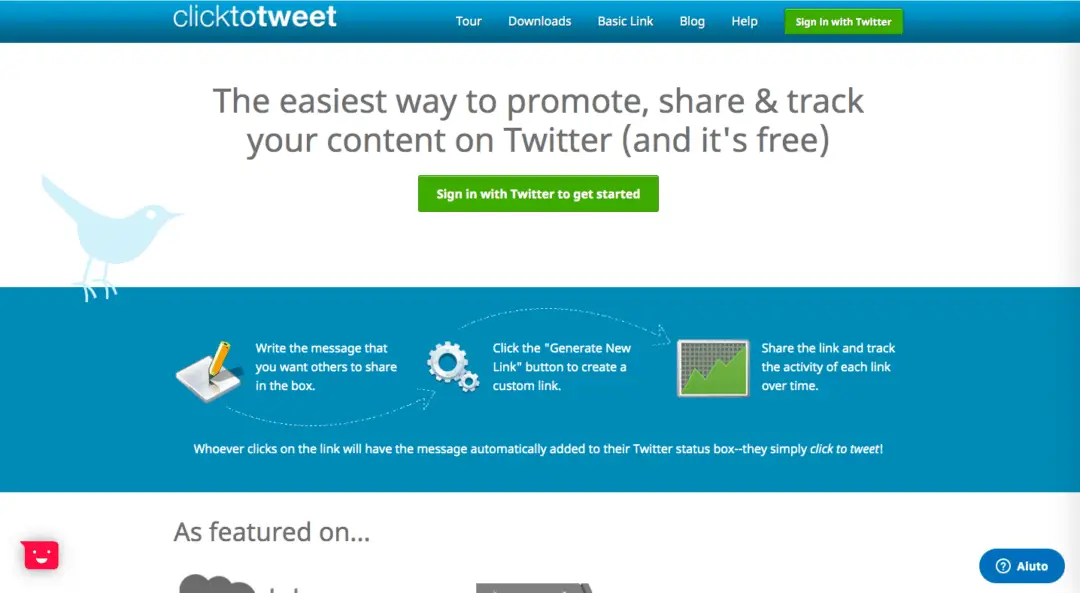In this image, we see a detailed screenshot of a website designed to promote and facilitate sharing content on Twitter. At the top of the page, there is a prominent blue banner featuring several navigation options in white text along the upper left corner, including "Click to Tweet." Moving from left to right, the menu includes tabs labeled "Tour," "Downloads," "Basic Link," "Blog," and "Help." On the right side of the banner, there is a green action button that says "Sign in with Twitter."

Below the banner, the background changes to a light blue shade adorned with a blue Twitter bird logo. The main header in this section reads: "The easiest way to promote, share, and track your content on Twitter—and it's free." Directly beneath this headline is another green action button, inviting users to "Sign in with Twitter to get started."

Further down, there is a blue box featuring instructional text on how to use the service. The instructions detail the process: write the message that you want others to share in the available text box, then click the "Generate New Link" button to create a custom link. Once created, share the link to track the activity generated by it over time. The explanation notes that anyone who clicks on the link will find the prewritten message automatically added to their Twitter status box, making it easy for them to simply click and tweet.